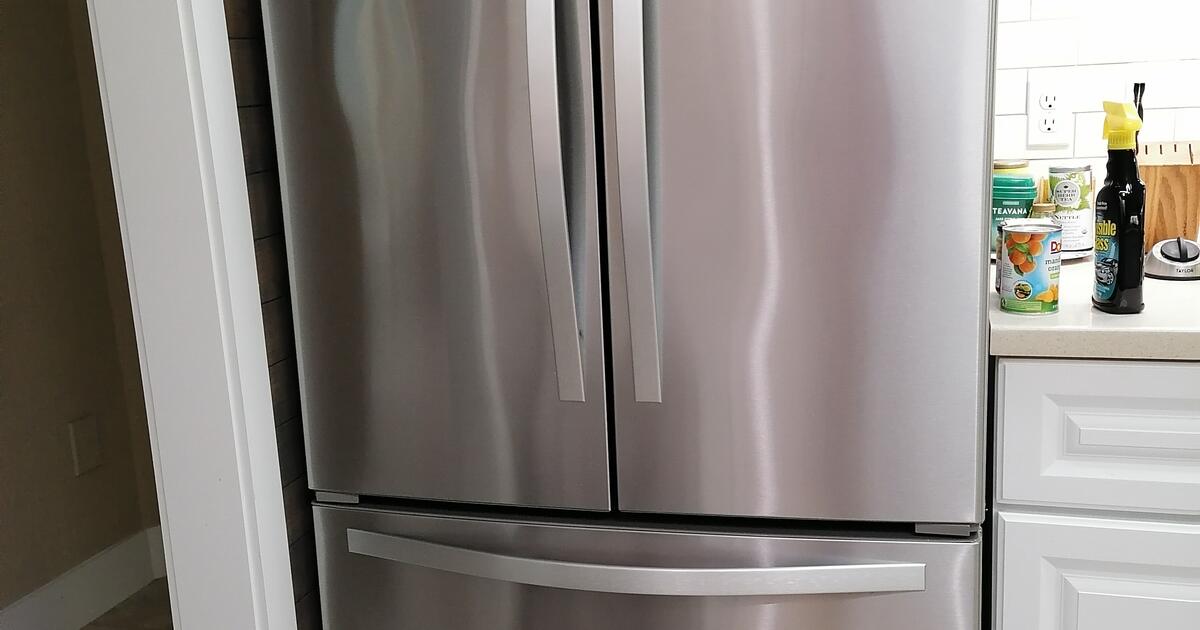The image features a modern kitchen setting, centered on a sleek, silver French door refrigerator with a bottom freezer. The refrigerator boasts flat handles and a minimalist design. To the left of the refrigerator is a white partition wall extending towards a hallway. The hallway wall is painted brown and includes an off-white electrical outlet with a white baseboard beneath it.

On the right side of the refrigerator, white cabinets line the space. Above these cabinets is a white light fixture mounted on a white tiled wall, providing a bright, clean look to the room. The countertop below the cabinets displays an assortment of kitchen items.

Prominently positioned is a can of Del Monte brand peaches, recognizable by its red "Del Monte" lettering and vivid imagery of peaches set against a blue background. Beside the can is a black bottle labeled "Invisible Glass" in prominent yellow letters, which sports a matching yellow cap.

Behind these items stands a black chalk square board adorned with slots typically used for knife storage. Directly in front of the board, on the countertop, is a small gray and black timer. The timer features a black dial that can be turned to set the desired time.

The overall scene captures a snapshot of a well-organized, functional kitchen space adorned with modern appliances and everyday kitchen essentials.